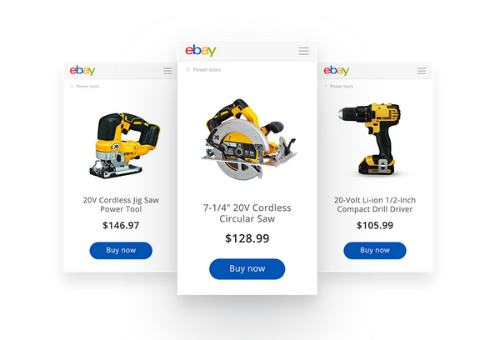In this eBay website screenshot, three distinct pop-up advertisements are prominently visible. The image showcases the familiar eBay logo in the top left corner, with 'e' in red, 'b' in blue, 'a' in yellow, and 'y' in green. The top right corner houses a light gray hamburger menu icon.

At the center of the screen, the highlighted pop-up features an image of a yellow and black circular saw, its metal blade gleaming in silver. The text below the image reads "7-1/4 20V Cordless Circular Saw," accompanied by a price tag of $128.99. A call-to-action bubble indicates "Buy Now."

To the right of this highlight, another pop-up advertises a "20V Lithium-Ion 1/2 Inch Compact Drill Driver," with a listed price of $105.99 and a "Buy Now" option.

On the far left, the final pop-up showcases a "20V Cordless Jigsaw Power Tool," priced at $146.97.